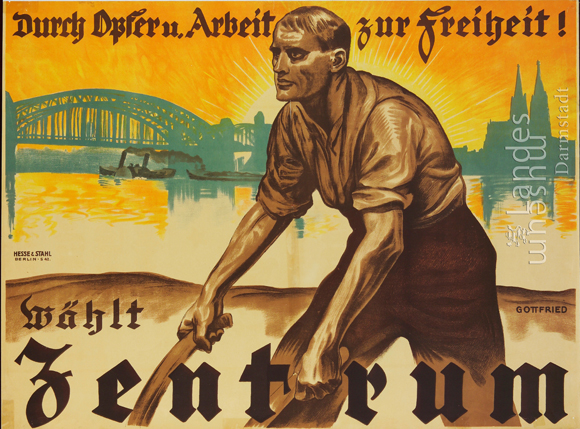The image is an intricately detailed illustration resembling a stamp, featuring a hard-working man at its center. The man, depicted with short blonde hair, wears a brown shirt with rolled-up sleeves and dark brown trousers. He is bent forward, gripping the handles of a wheelbarrow or plow as if engaged in intense labor, with his gaze directed upwards to the left. The background showcases an orange sky with the emerging yellow sun casting rays, evoking an evening sunset. To the left, an arched, steel bridge stands in silhouette, reminiscent of the Golden Gate Bridge. The right side of the background features silhouetted skyscrapers or towers, possibly with spires, suggesting a cityscape. Below, there's a body of water reflecting the vibrant sky, where steamboats with smokestacks sail. The foreground displays brown soil or ground where the man stands. The top of the image contains text in a classical, medieval-style font, possibly in German, reading "Döri, Döfri, Arbeit zur Freiheit." Additional text at the bottom states "Walt Zentrum," with "Landesmuseum" written vertically in white or light grey on the right side. The entire composition suggests a theme of labor and perseverance amidst an urban setting.